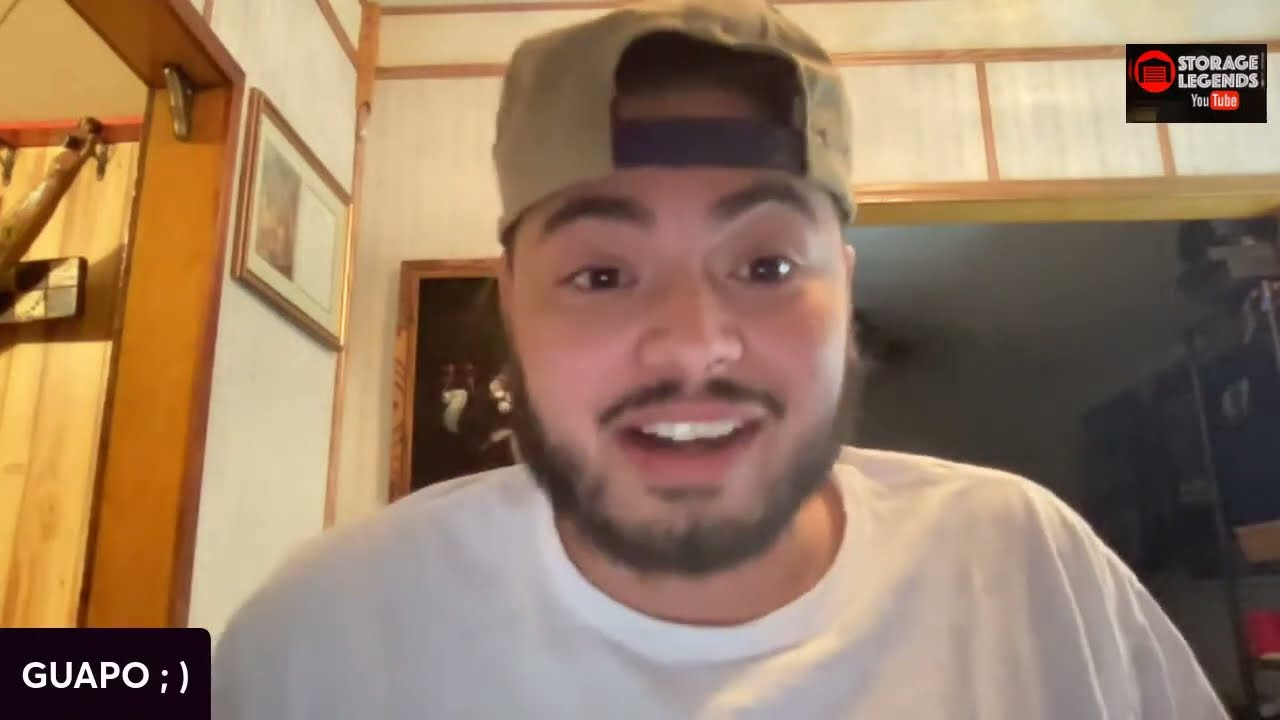The image captures a man with an expression that is a mix of a smile and surprise, wearing a plain white T-shirt and a tan baseball cap worn backwards. He has an unkempt beard, includes a mustache and a goatee. His white teeth are prominently visible as he faces the camera. He appears to be in a living room, characterized by light brown walls with dark brown trim and an opening to another room in the background. On one wall behind him, there is a large painting, possibly of Jesus on the cross. The lower left corner of the image features a small black rectangle with the word "guapo;" followed by a winking smiley face, indicating the word "handsome" in Spanish. The upper right-hand corner displays a logo that reads "Storage Legends," with "YouTube" beneath it, along with a red trademark circle.